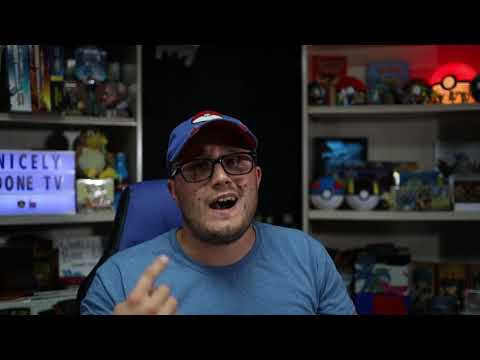A Caucasian man with black-framed glasses sits at the center of the image, his face marked by slight blemishes and beard stubble. He's wearing a blue t-shirt and a blue baseball cap featuring a red and white Poké Ball on it. His left hand gestures near his face, indicating he might be passionately explaining something, with an intense expression possibly suggesting animated discussion or reacting to a comment. Behind him, there's a high-end gamer chair with a visible blue backrest and two large, cluttered shelves flanking either side. Both shelves are brimming with Pokémon merchandise, including various colored Poké Balls, toys, and board games. Notably, on the right shelf's top tier, a glowing red and white Poké Ball lamp illuminates the scene, adding a striking touch. The left shelf also holds a mix of memorabilia and books, including comic books and hardcovers. A lit-up sign reading "Nicely Done TV" is prominently displayed, further indicating this might be a well-known Pokémon-themed streaming setup.